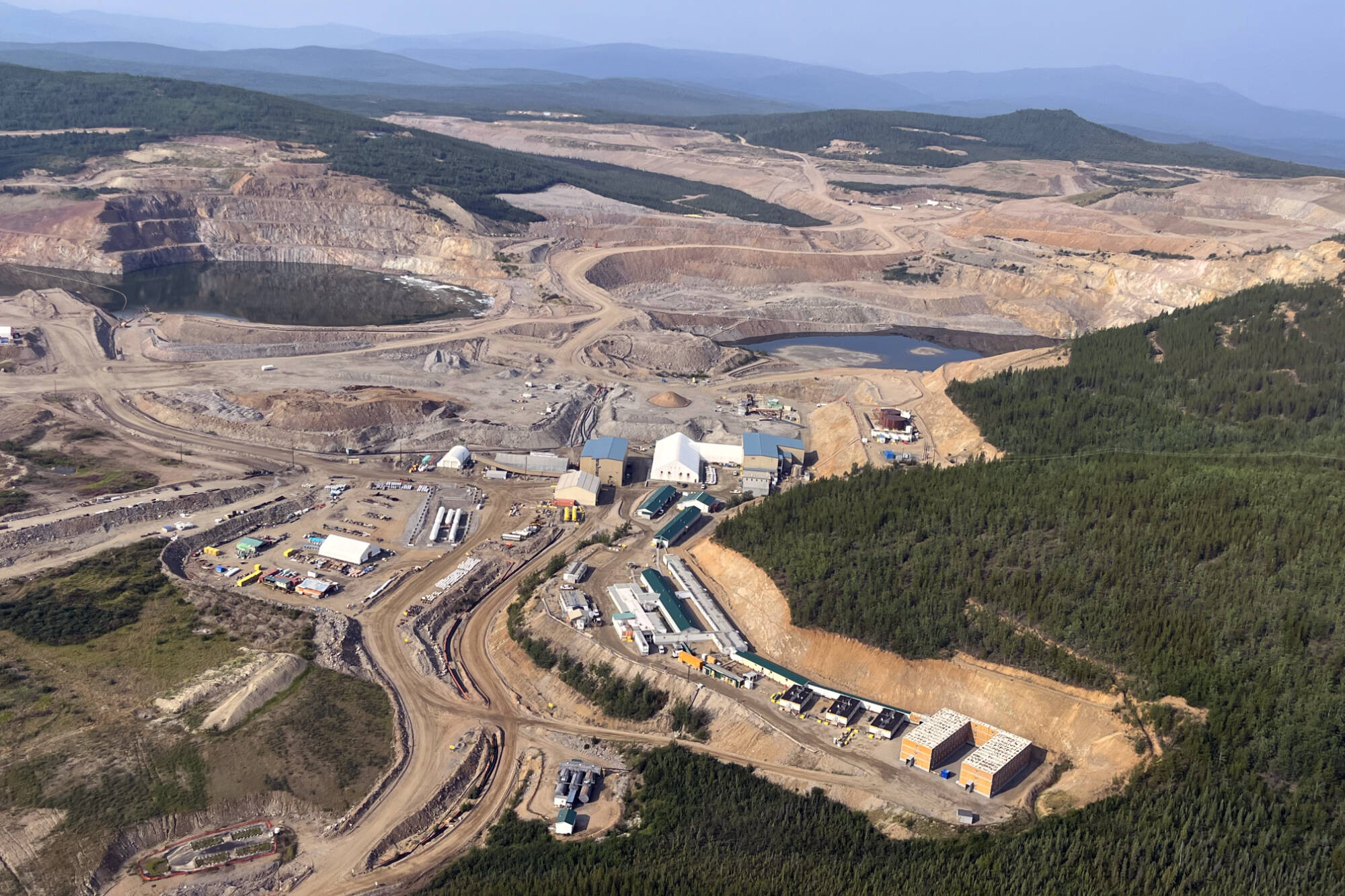The image is an aerial photograph showcasing a mining complex amidst a wilderness setting. The shot appears to be taken from a significant height, possibly from a drone or plane, revealing a large expanse of earth. Dominating the lower right area is a dense forest, possibly of evergreen trees, indicated by their dark, textured appearance. This forest transitions into the middle section where the mining operations begin. The mining complex itself features numerous pits and holes, areas of dug-up, grey-tan soil, and some low-lying construction buildings, suggesting an ongoing development, possibly an airport or another major infrastructure project. In the upper left corner of the photo stands a vertical rock formation resembling a canyon carved by water, adding to the rugged terrain. The sky above is a light, smoky blue, indicating a hazy atmosphere. Finally, amidst this expanse is a body of dark blue water, contributing to the varied landscape captured in this detailed aerial view.